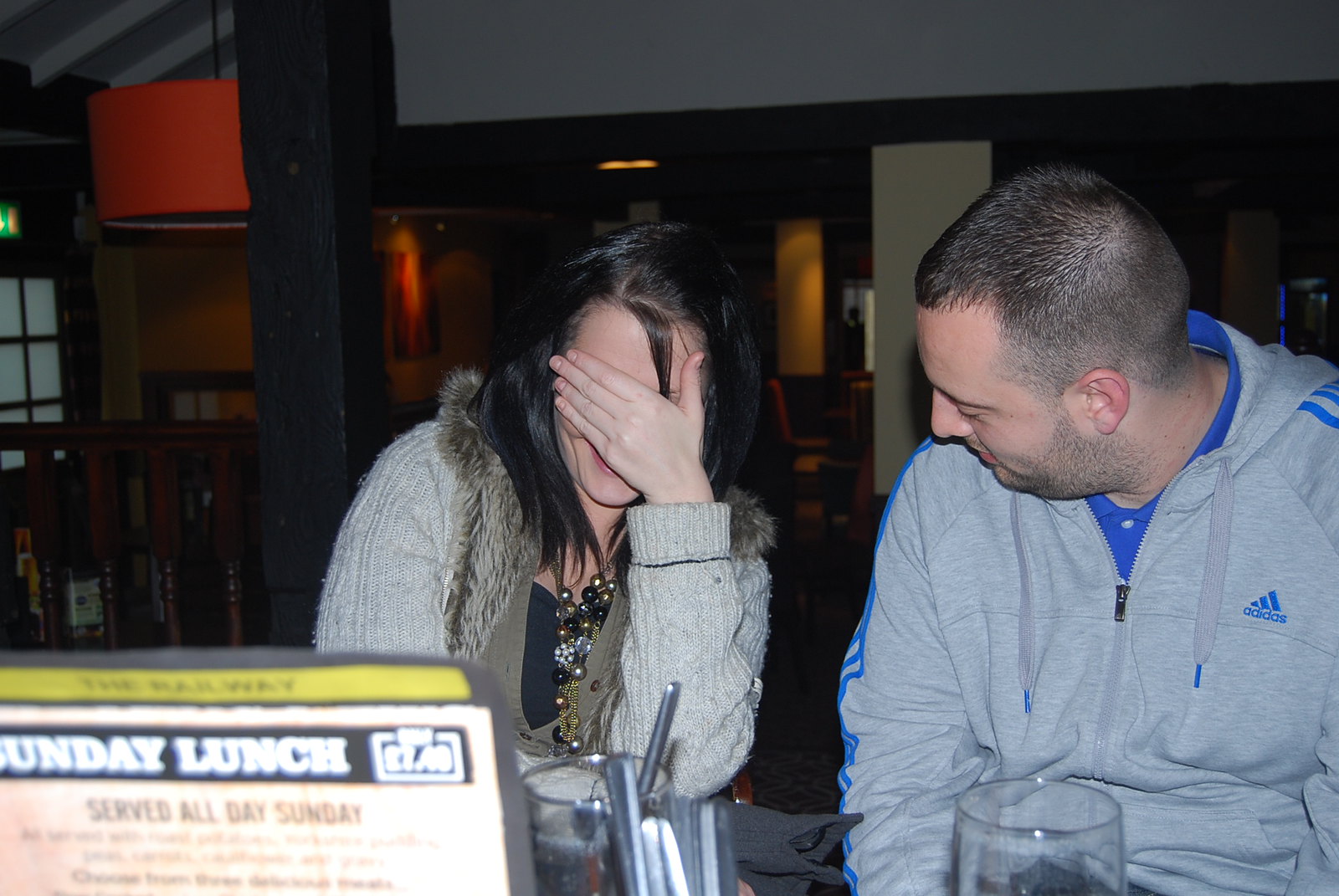This photograph captures a moment inside a dimly lit pub featuring a man and a woman seated at a table. The woman, positioned on the left, has long black hair and is wearing a light grey knit jacket adorned with fake fur around the collar. Underneath, she has on a black shirt, paired with a beaded necklace comprising black, gold, silver, and pearl elements. Her left hand covers her face, partially revealing a smile that suggests she is laughing. The man on the right is observing her with a gentle expression. He has short, cropped black hair and a neatly trimmed beard. His attire includes a grey hooded Adidas sweatshirt with blue stripes down the sleeves, layered over a blue collared shirt. Both are sitting with empty glasses and silverware in cups before them, indicating they may have finished a meal. In the lower left corner, a menu card stating "Sunday lunch, served all day Sunday" can be noticed. The background reveals elements of the pub's interior such as wooden hand railings, chairs, and lights, with some reflections captured from the camera flash.